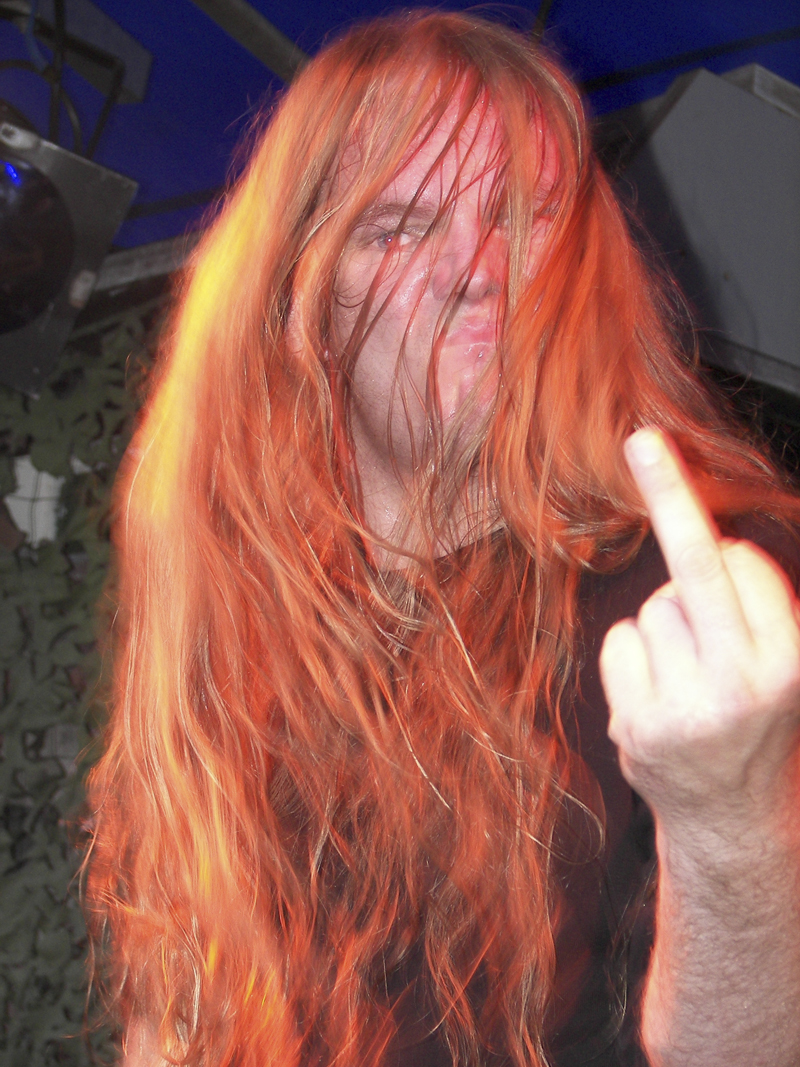This full-color photograph captures a striking image of a musician with waist-length, vividly bright red hair, illuminated dramatically with a shine. The subject's hair, appearing somewhat messy with multiple strands falling across his face, leaves only one blue eye visible. The intense, angry expression on his face is accentuated by the glare in his eye, giving it a red tint. He is wearing a short-sleeved black top and making an obscene gesture with his left hand, prominently displaying his middle finger. The backdrop features a dark, almost black sky tinged with dark blue hues, suggesting it was taken either indoors or at night. Additionally, there are stage lights, framed by metal and wires, positioned above him with a distinct blue light that isn't turned on. The setting evokes a concert atmosphere, emphasizing the artist's rebellious and intense persona. The photo is devoid of any text, date, or name.